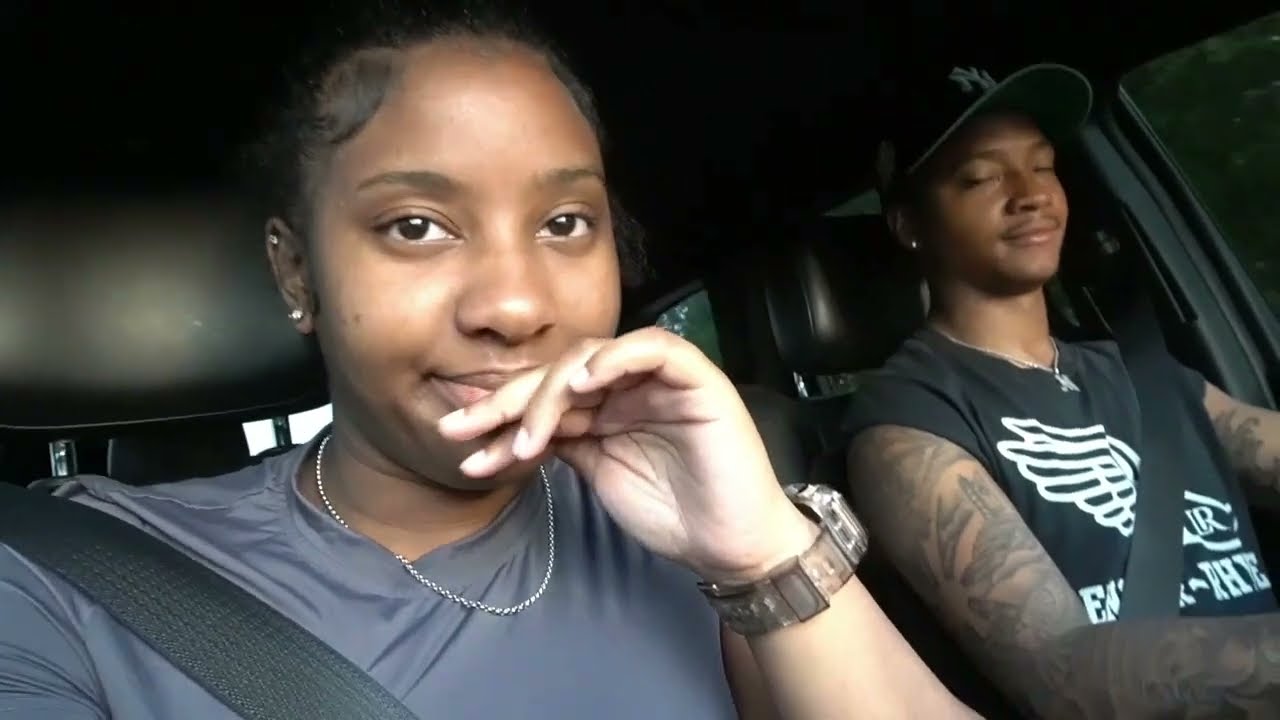This horizontally-oriented, color photograph captures an intimate moment inside a vehicle, showcasing two young African-American individuals. The young woman in the passenger seat, likely the photographer, is taking a selfie. She is in her late teens or early 20s, wearing a gray shirt, a silver chain necklace, and an Apple or fitness watch on her left wrist. Her short black hair is pulled back, revealing two earrings on her right ear. She gazes at the camera with her left hand resting against her closed mouth, emphasizing her contemplative brown eyes.

Seated to her right, the young man is driving, exuding a relaxed demeanor with his eyes closed and a slight grin. He sports a sleeveless black tank top adorned with a white design resembling an eagle's wing, and a black New York Yankees ball cap with white lettering. His heavily tattooed arms add an intricate layer of detail to the image, and he also wears a silver neck chain. His right shoulder is secured by a gray seatbelt strap. The photograph focuses on the occupants while the dark interior of the vehicle forms an unobtrusive backdrop, emphasizing the connection and shared moment between the two.